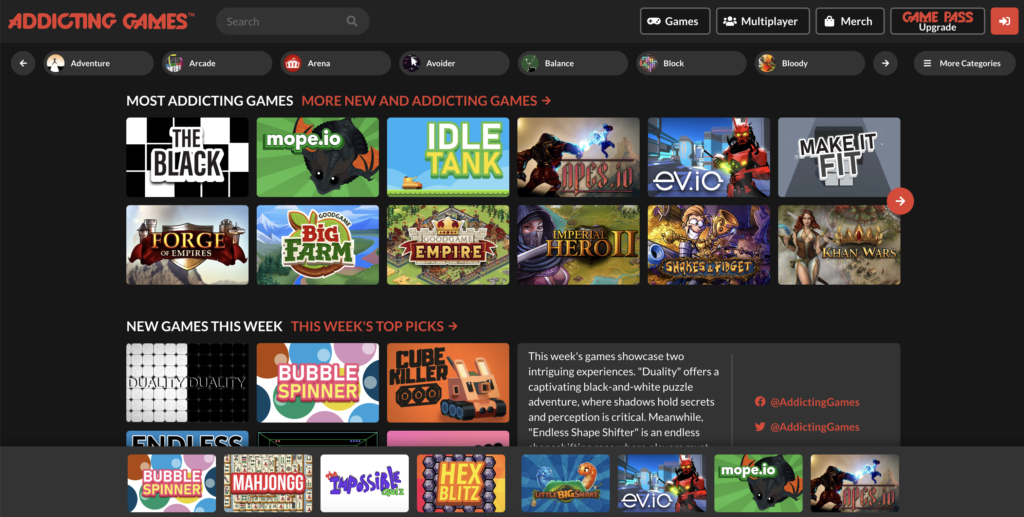This detailed screenshot appears to be from a website, likely Addicting Games, based on its layout and visual elements. The image features the Addicting Games logo prominently in the upper left corner, displayed with orange text in capital letters, styled with a curved and rounded font. This logo is set against a dark grey banner that spans the top of the image.

Adjacent to the logo is a search bar, flanked by several tabs titled Games, Multiplayer, Merch, Game Pass, and Upgrade, suggesting navigational options for the user. Below this banner is a series of clickable game category labels encapsulated in small grey ovals. These categories include Adventure, Arcade, Arena, Balance, Block, and Bloody, with navigational arrows on either side indicating more options are available.

Beneath the category labels are two rows of game thumbnails, each row containing six images. The visible games include The Black, Idle Tank, Make It Fit, Big Farm, and Imperial Hero 2, among others, with additional selections visible beneath these rows.

The overall background of the screenshot is predominantly black or dark, which contrasts with the grey elements and colorful game thumbnails, making the layout user-friendly and visually engaging.